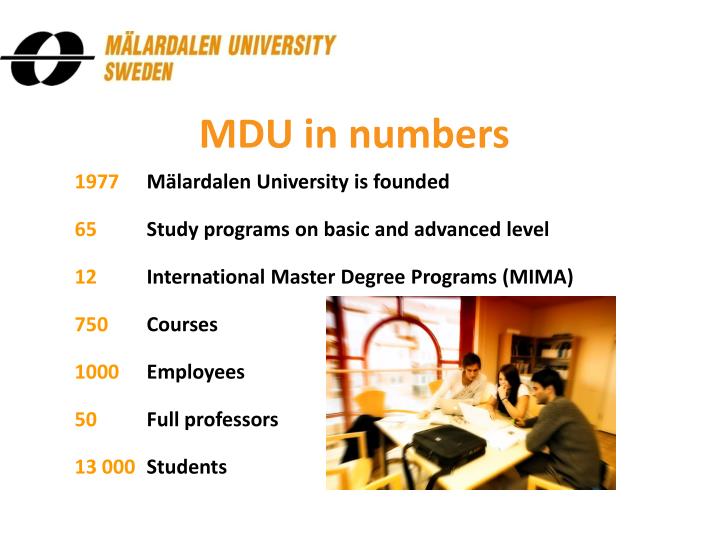The image is a PowerPoint presentation slide detailing key statistics about Mälardalen University, Sweden. At the top left, there is a distinctive black logo consisting of two interlocking circles with a horizontal line intersecting them. To the right of the logo, in bold orange text, it reads "Mälardalen University, Sweden." Directly beneath this heading, a section titled "MDU in numbers" enumerates significant data about the university. 

Highlighted in gold and black text are several key statistics: 
- Founded in 1977
- 65 study programs at both basic and advanced levels
- 12 international master's degree programs
- 750 courses
- 1,000 employees
- 50 full professors
- 13,000 students

In the bottom right quadrant of the slide, there is a photograph depicting three students working together at a light-colored table, with books and a green-and-black object visible. They are situated near a window, enhancing the natural light in the scene, with the setting blending harmoniously with the slide's brown and yellow color scheme.